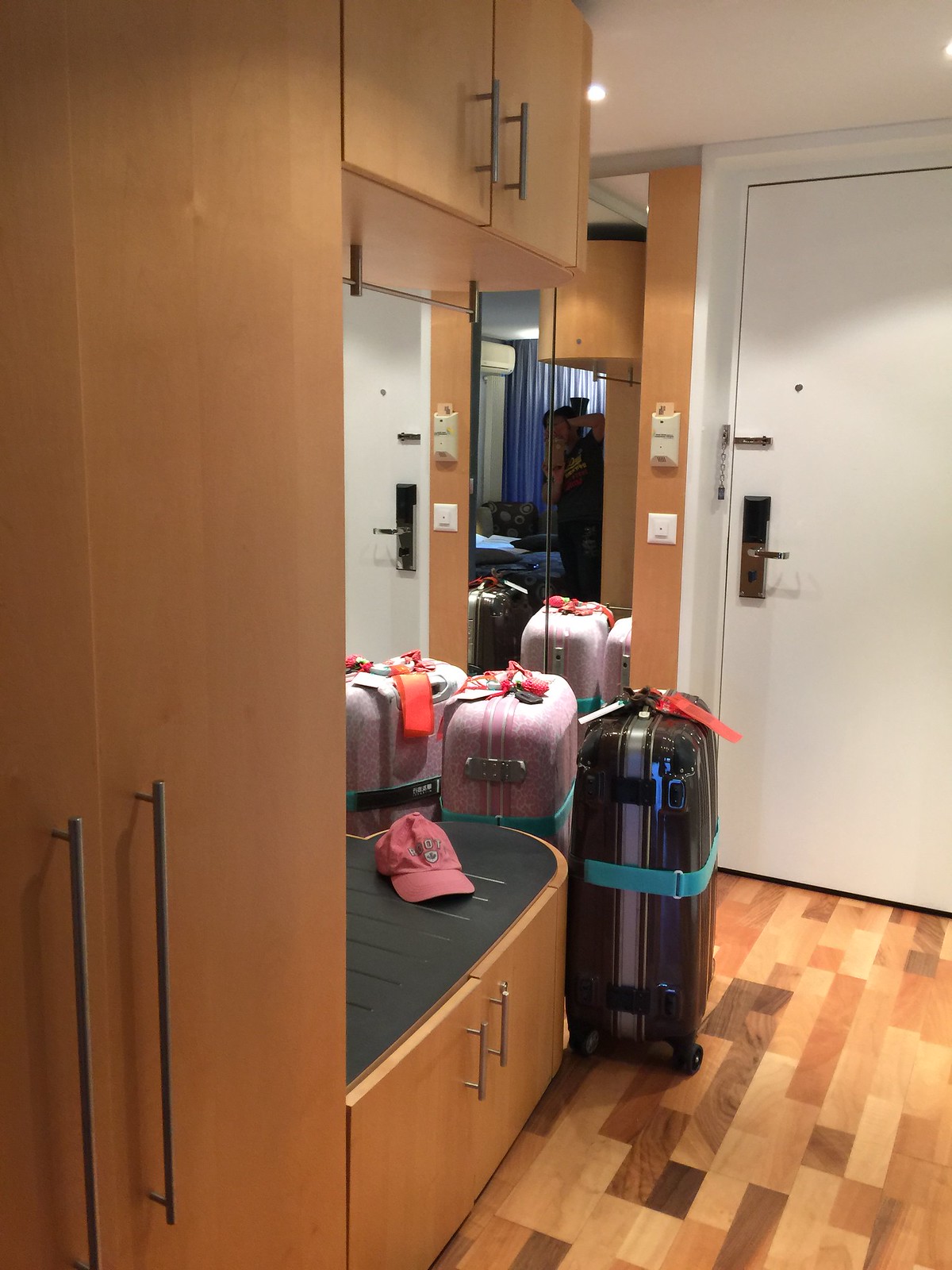The photograph captures the interior of what appears to be a small hotel room, featuring a mix of modern amenities and vibrant colors. Visible in the center of the image is a closed white door with standard hotel locks. Directly in front of the door, there are three suitcases arranged upright, the most prominent of which are a black suitcase with a distinctive blue band around its middle and a pink suitcase similarly accented with a blue band. A third suitcase, white with a red tag, is partially visible. 

To the left of the suitcases, a wooden cabinet stretches from the floor to the ceiling, integrating various storage solutions. This cabinet includes upper and lower compartments, a central bench, and a mirror that reflects both the suitcases and the door. The central bench also serves as a seating area, atop which rests a pink baseball cap, adding a splash of color to the setting. Adjacent to this arrangement is a large wardrobe with long handles, enhancing the room's storage capacity.

The multicolored hardwood floor, likely a thick wooden tile designed to imitate real wood, adds warmth and contrast to the room's overall décor. The background includes a brown wall that complements the wood and gives a cozy feel to the room. Overall, the image showcases a well-organized, compact living space characteristic of modern hotel rooms.